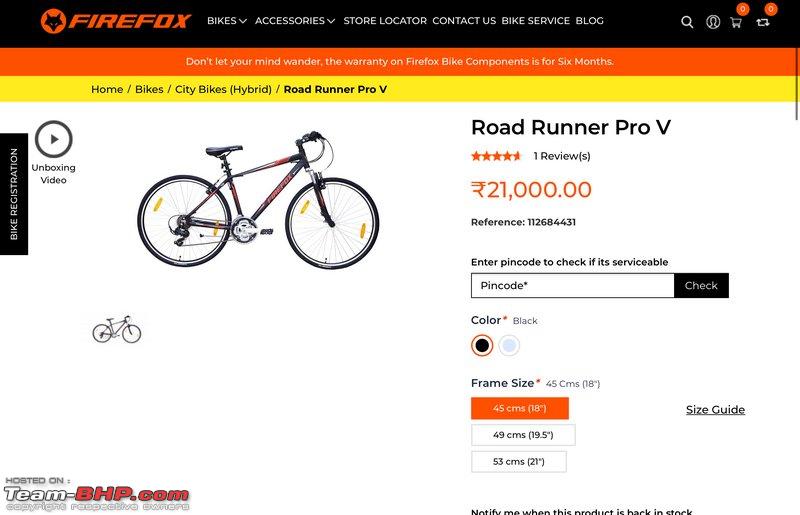The screenshot showcases a webpage from the Firefox Biking Company, a purveyor of bicycles and bicycle accessories. At the top of the page, the company's branding is prominently displayed with the Firefox logo—an elegant, all-black fox silhouette set against a striking orange circle. The company name "FIREFOX" is rendered in bold, orange uppercase letters, all on a sleek black background. Adjacent to the logo, navigation options are clearly listed: Bikes, Accessories, Store Locator, Contact Us, Bike Service, and Blog. Additionally, user interface icons for Account, Shopping Cart, and Search are also visible.

The main focus of the page is a highlighted product, a mountain bike named "Roadrunner Pro-V." The left side of the page features a detailed image of this standard mountain bike, characterized by its large wheels. To the right of the image, the product details are elaborated: the bike has earned a rating of four and a half stars based on one review, and is priced at $21,000 in an unspecified currency. The selected frame size for the bike is 45 centimeters, marked in orange to indicate selection, and the chosen color is black.

At the bottom of the screenshot, a discreet watermark reads "hosted on team-bhp.com," indicating the hosting website.